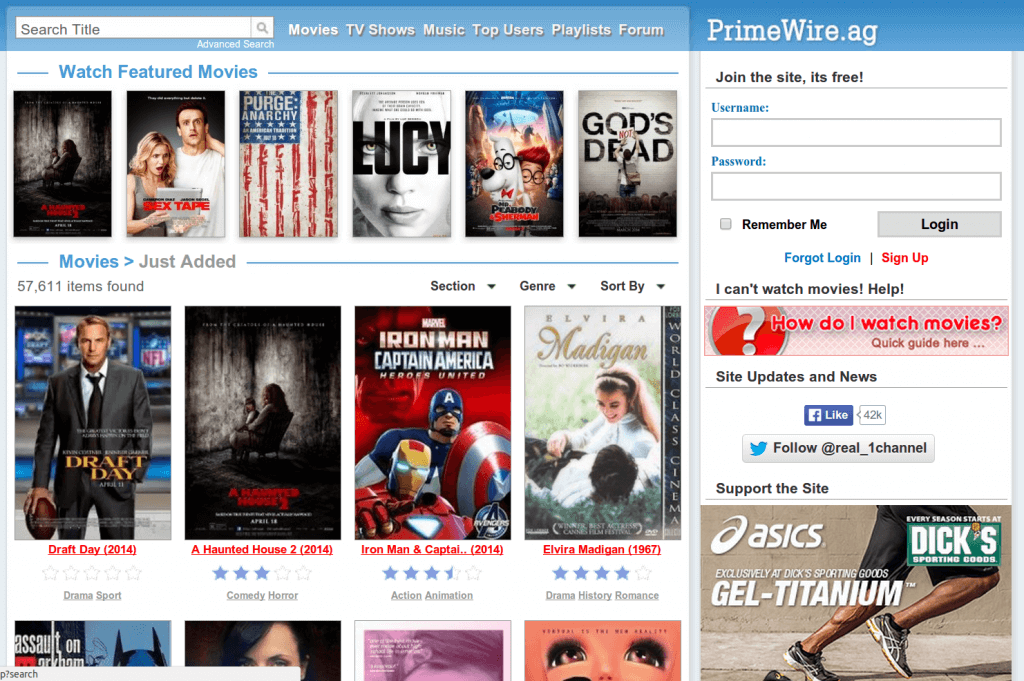The image depicts a comprehensive and detailed interface of a media website named "Promwire.ag." At the top, there's a search bar followed by categorized navigation options including Movies, TV Shows, Music, Top Users, and a section for Playlists.

There are prominent calls to action encouraging users to join the site for free. Users can input their Username and Password into designated boxes, with options to "Remember Me" and "Log In." For further convenience, there is also an advanced search feature available.

The homepage showcases a "Watch Featured Movies" section displaying six films. Specific titles visible include "Sex Tape," "The Purge: Anarchy," "Lucy," and "God's Not Dead." Additionally, the site boasts an impressive library with "57,611 items found" under the "Movies Just Added" section.

A genre selection tool and a sort bar facilitate user navigation. Another set of four highlighted movies includes "Draft Day," "A Haunted House 2," with "Iron Man," "Captain America," and what appears to be "Madigan" listed next. The movies are accompanied by user ratings: the first movie has no stars, the second movie has three stars, the third has three and a half stars, and the last movie boasts four stars.

On the right side of the interface, there are quick links for "Forgot Login" in blue and "Sign Up" in red. Additionally, there is a "Help" section addressing issues like "I Can't Watch Movies" for user support.